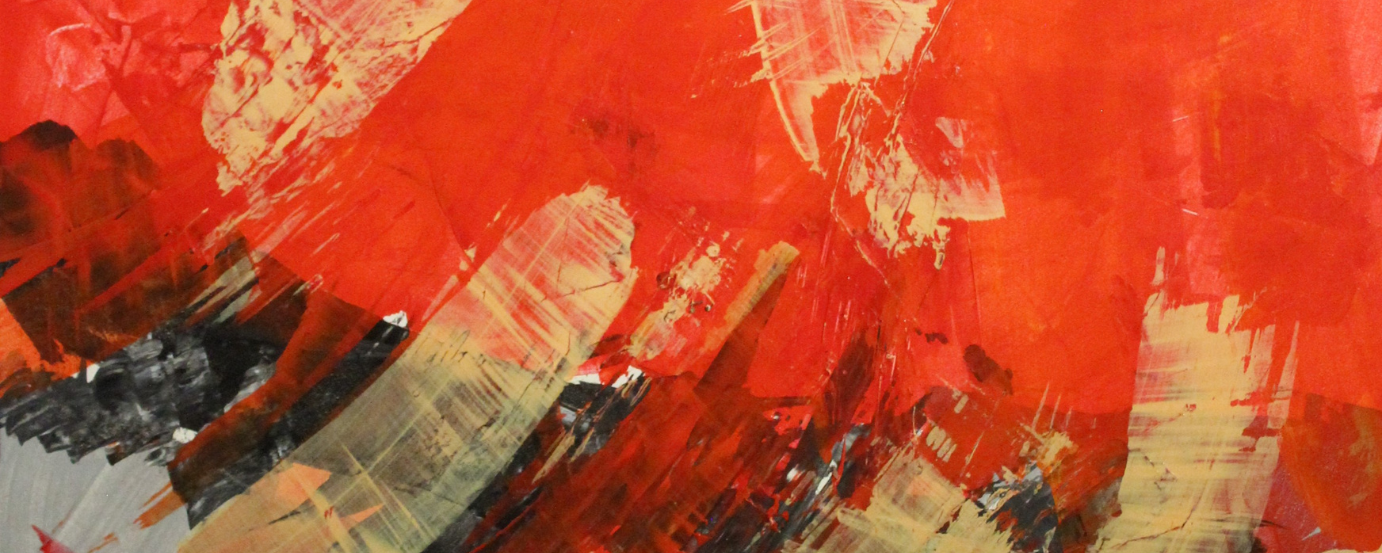The image is an abstract painting characterized by a horizontal and thin orientation. The dominant color is red, primarily concentrated in the upper section and extending down the right side. These red hues are complemented by mixed gold and yellow tones, creating vertical-like features reminiscent of buildings. Swooshes of dark and light gray, peach, pink, and cream add complexity and texture, with gray predominantly concentrated at the bottom and left side of the painting. The bottom section also includes dark, almost black tones melded with white, orange, and tan. The work is a dynamic composition of colors and textures, devoid of any tangible forms, highlighting the emphasis on abstraction through a harmonious yet chaotic blend of hues.